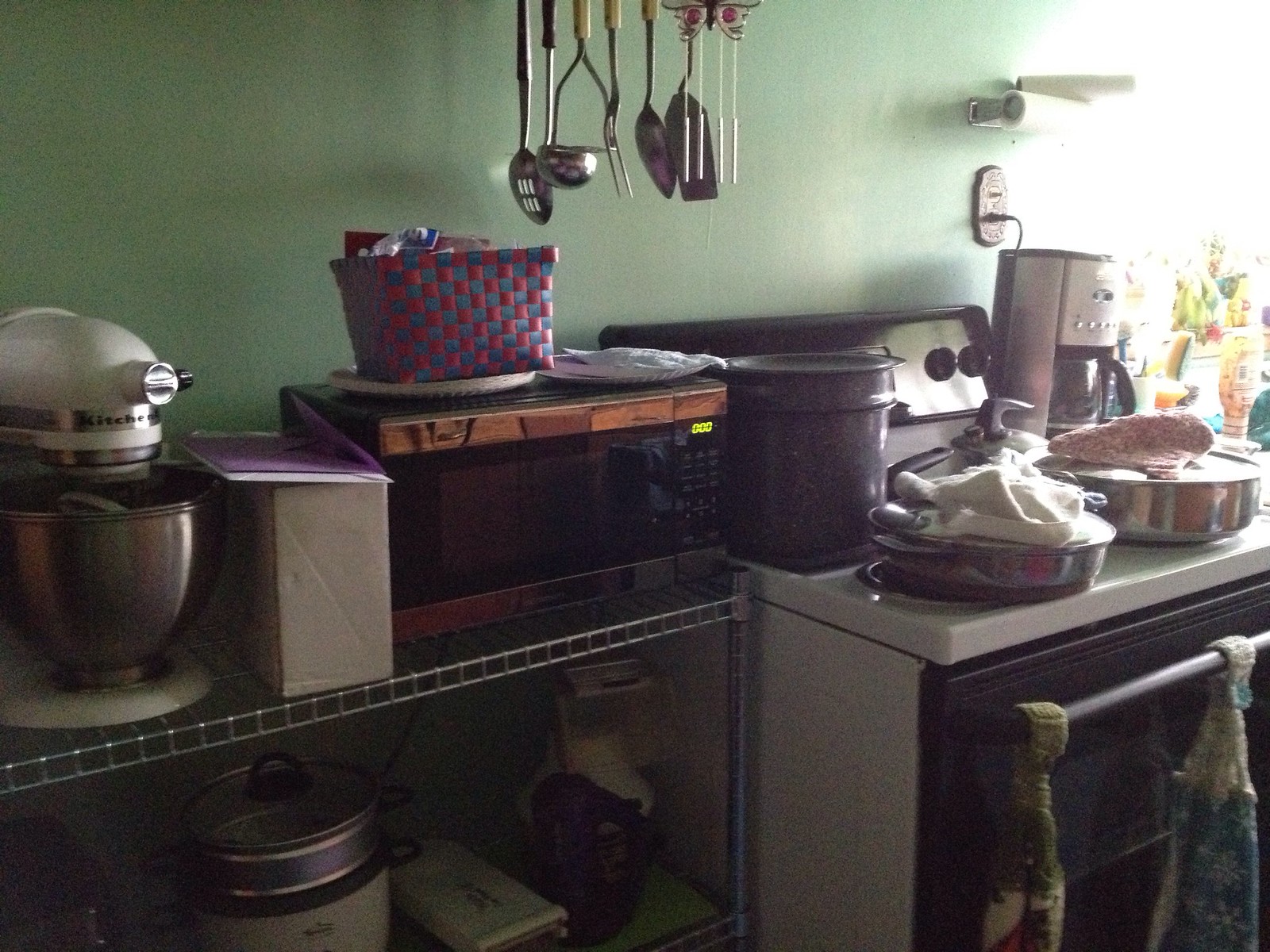The image depicts a somewhat cluttered kitchen with a light green wall as the backdrop. Various utensils hang from the underside of a cabinet, accompanied by a whimsical, white butterfly adorned with red highlights, and a small chime with dangling silver elements positioned above the utensils. 

On the wall, there's a mounted paper towel holder and a visible electrical outlet to which a silver-fronted coffee maker is plugged in. The white stove, featuring a black front, has two multicolored green and brown towels draped around its oven pull bar. On the stovetop, two silver skillets are covered with cloths—one with a pinkish pot holder and the other with a white towel. A large black stock pot sits towards the rear.

Natural light floods through a window positioned above the sink, illuminating the scene and highlighting an assortment of plants and bottles placed on the windowsill. To the far side of the stove, there's a wire shelving rack holding a small black microwave. On the shelf above the microwave rests a vibrant red and blue basket, a large silver mixer, and a white box, with various canisters and items stored on the lower shelves. The overall scene captures the lived-in and eclectic essence of the kitchen space.